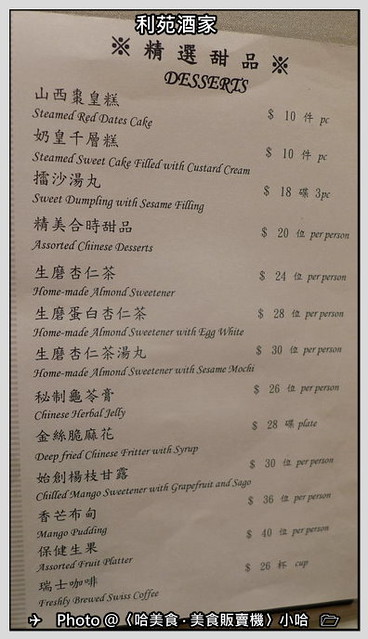This color photograph captures a detailed dessert menu featuring both an Asian language and English translations. The heading at the top of the menu is labeled "Desserts," and each item is presented with Asian characters above the English descriptions. The menu includes the following items and prices:

- Steamed Red Dates Cake - $10
- Steamed Sweet Cake Filled with Custard Cream - $10
- Sweet Dumpling with Sesame Filling - $18 for three pieces
- Assorted Chinese Desserts - $20 per person
- Homemade Almond Sweetener - $24 per person
- Homemade Almond Sweetener with Egg White - $28 per person
- Homemade Almond Sweetener with Sesame Mochi - $30 per person
- Chinese Herbal Jelly - $26 per person
- Deep Fried Chinese Fritter with Syrup - $28 per plate
- Chilled Mango Sweetener with Grapefruit and Sago - $30 per person
- Mango Pudding - $36 per person
- Assorted Fruit Platter - $40 per person
- Freshly Brewed Swiss Coffee - $26 per cup

At the bottom of the menu, there is a note that reads "Photo At" followed by some Chinese lettering. The menu is vibrant and clearly laid out, making it easy to navigate the diverse selection of traditional and contemporary Chinese desserts.